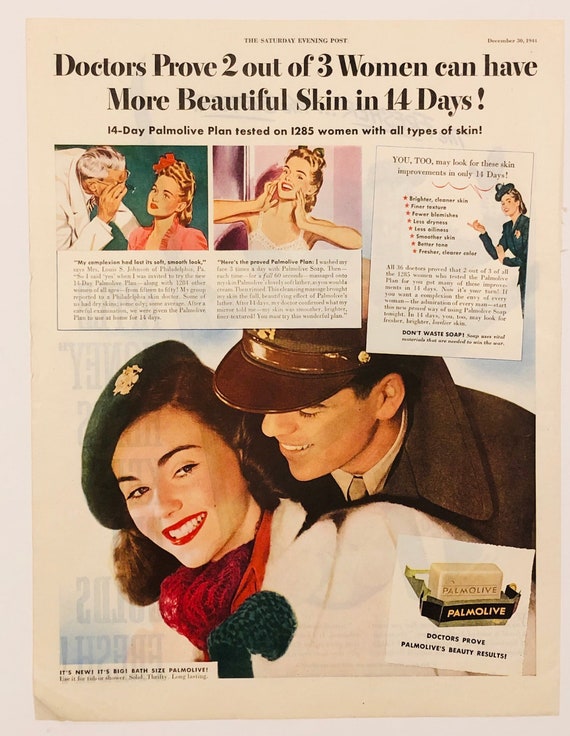This is a vintage advertisement, featured in the December 1944 issue of the Saturday Evening Post, promoting Palmolive soap. The headline boldly proclaims, "Doctors prove 2 out of 3 women can have more beautiful skin in 14 days," highlighting a 14-day Palmolive plan that was tested on 1,285 women with various skin types.

The ad comprises several images: a doctor examining a woman's facial skin, the same woman later smiling and touching her cheeks with both hands in delight, and another woman pointing out the benefits of using Palmolive soap. These smaller images are laid over a larger central image featuring an ecstatic woman in a white coat, black beret, and red scarf, smiling to her left. Behind her stands a smiling man wearing a brown winter jacket and hat, looking fondly at her.

In the bottom right corner, an image of a Palmolive soap bar is accompanied by the caption, "Doctors prove Palmolive's beauty results." This detailed and visually compelling layout aims to convey the effectiveness and trustworthiness of Palmolive soap in enhancing women's skin beauty.